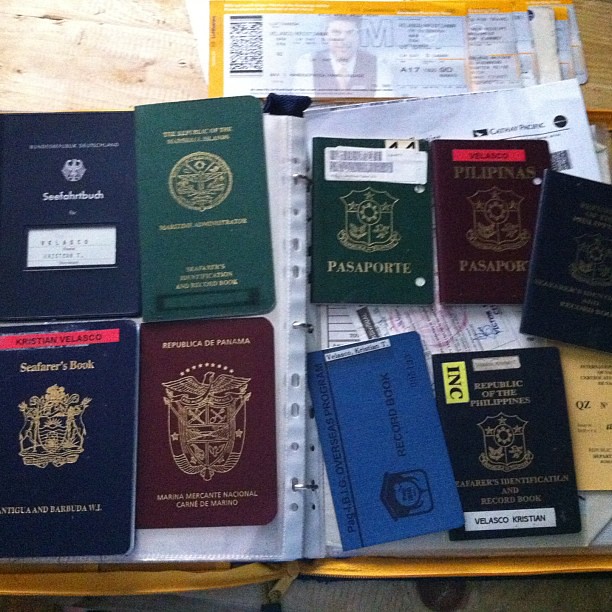Captured from a top-down perspective, this rich and detailed photograph showcases a diverse array of passports, meticulously arranged on a woodgrain table. The passports hail from various countries, featuring colors such as dark blue, green, maroon, royal blue, and burgundy. Visible passports include the Republic of the Philippines, Republic de Panama, and other identifiable documents, alongside an assortment of other indistinct passports that add to the international flavor of the display. 

In the background, a three-ring binder, left open, contains organized documents. To the left of the binder page, we spot two dark blue and green passports on the top, and a dark blue and burgundy passport below them. On the right-hand side, three passports—dark green, burgundy, and dark blue—sit above a royal blue and dark green passport.

Further details reveal a spiral notebook holding display pages for photos or papers, and a notable document with the Canadian Pacific railroad logo in the upper right corner is visible underneath. Among the passports, a navy blue one inscribed with NIC, Republic of the Philippines stands out. Adjacent documents include a light blue Page Overseas Programme record book, a maroon Republic de Panama passport, and other variously colored passports, some with blurry text and images, adding to the vivid and eclectic nature of the scene. The collective arrangement of these passport books and documents on the woodgrain table creates a compelling tableau of global travel and identification.